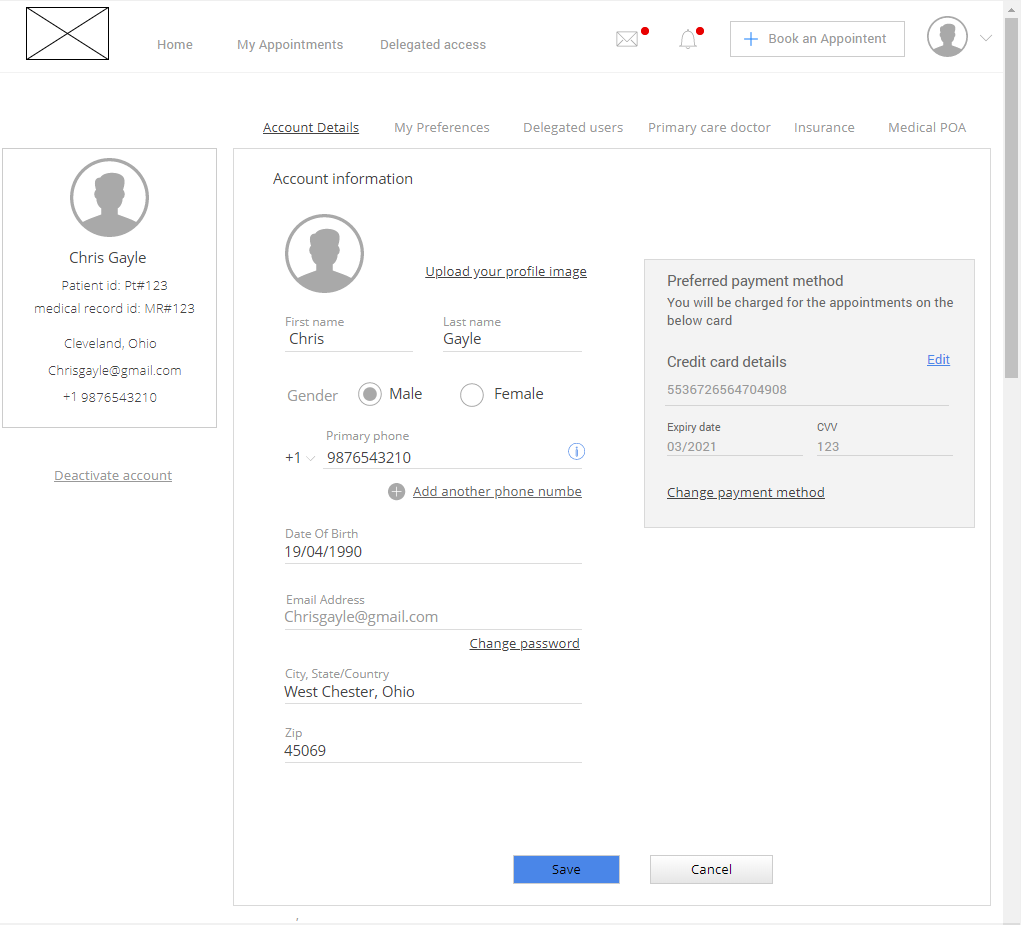This digital interface screenshot features a user account page for "Chris Gale." At the top of the page, there are navigation options including "Home," "My Appointments," and "Delegated Access." Prominently displayed is a "Book Appointment" button. The profile section for Chris Gale includes an email address and an option to upload a profile image. There's also a link to deactivate the account.

The payment information section specifies the preferred payment method, indicating that charges for appointments will be billed to the credit card ending in 1234 with an expiration date of March 2021. Users are given the option to change their payment method via a dedicated link. The interface includes a "Save" button for saving changes and a gray "Cancel" button at the bottom of the screen for discarding changes.

The layout is designed for user convenience, making it easy to navigate through account settings and manage appointments and payment methods.